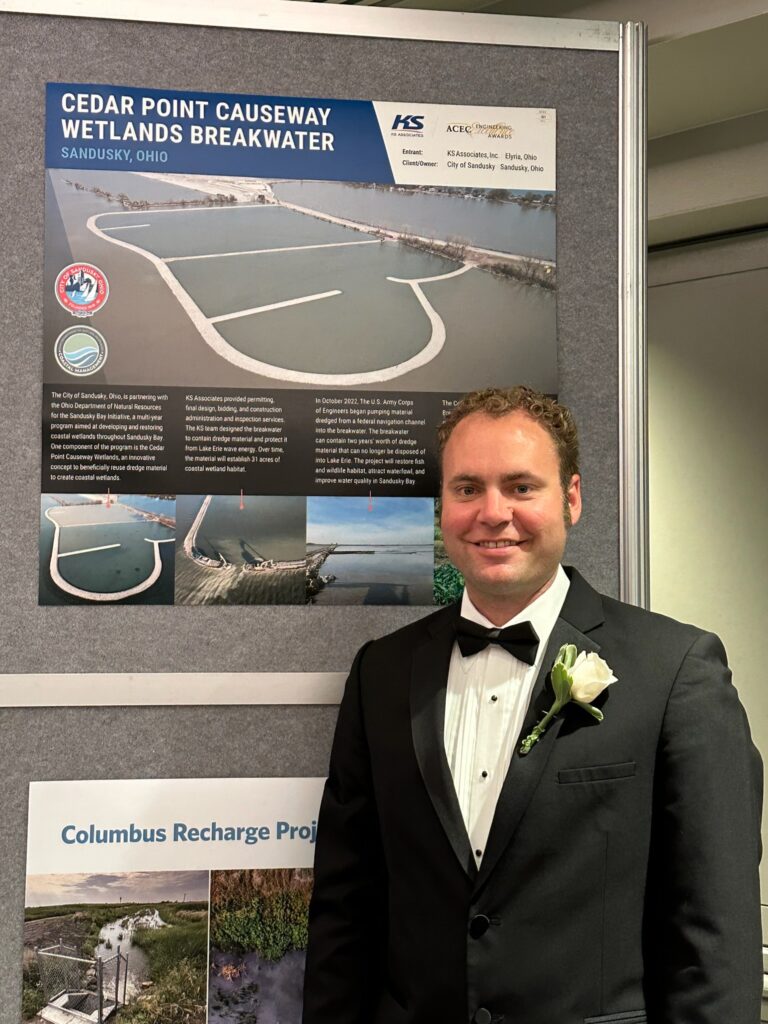This image features a smiling Caucasian man with curly brown hair, dressed impeccably in a tuxedo suit with a black bow tie and a white rose boutonniere on his lapel. The man appears to be in his forties and is standing in front of a gray display board resembling something you might find in an office setting. On the board, there are two prominent posters. The first one reads "Cedar Point Causeway Wetlands Breakwater, Sandusky, Ohio," accompanied by a photo likely depicting this causeway. The second poster, partially obstructed, mentions the "Columbus Recharge Project" and appears to feature images of bodies of water. The man's cheerful expression and formal attire suggest he might be attending a formal event or have some connection to the displayed projects.